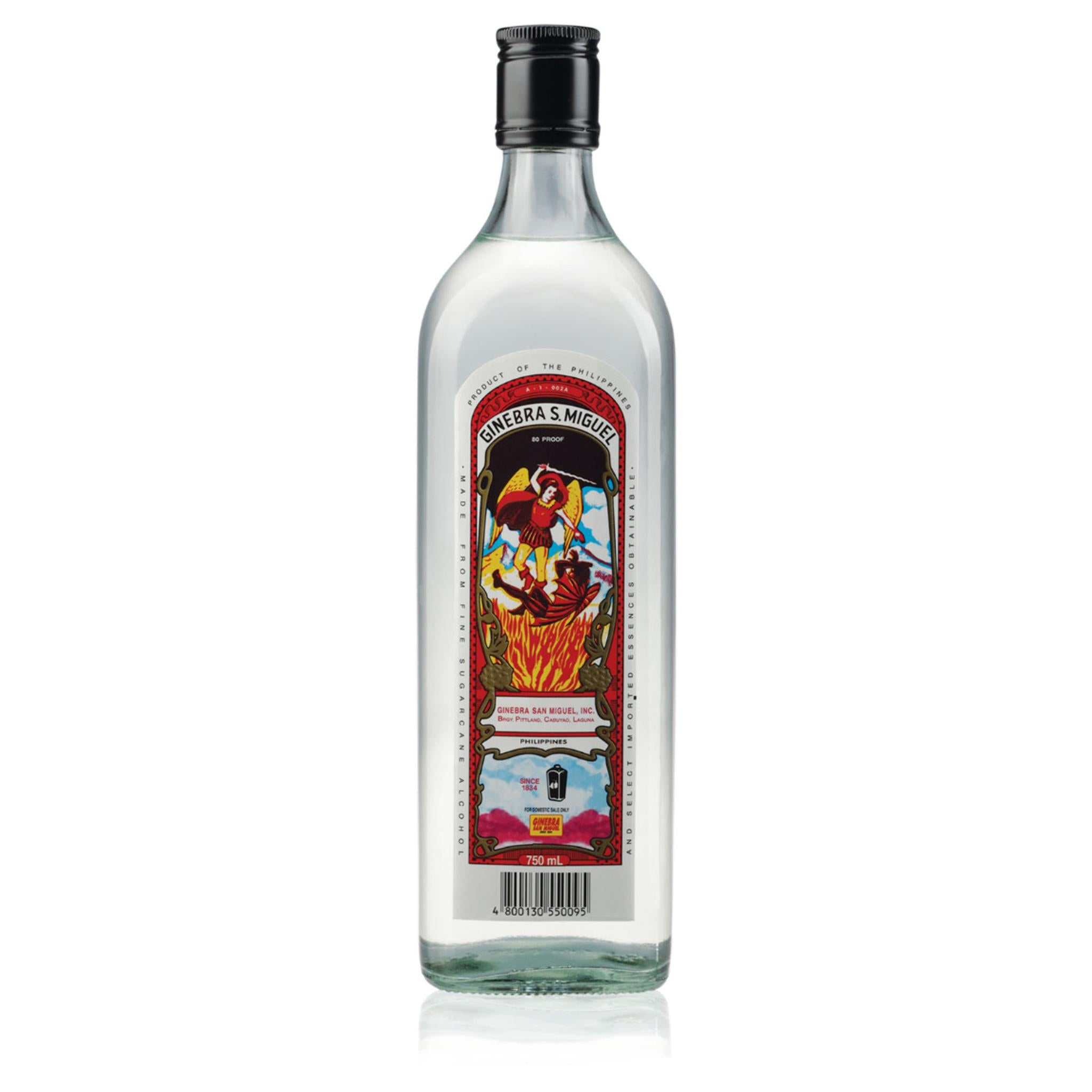The image portrays a 750 milliliter bottle of clear liquor, specifically Ginebra San Miguel, a product of the Philippines. This tall, slender glass bottle features a black twist-off screw cap. The front label, prominently red with a long rectangular shape and a rounded top, depicts a dramatic scene: a man donned in yellow tights, red boots, and a red outfit with goldish-yellow wings holds a sword, seemingly having vanquished a devil-like creature that is falling into a sea of flames. The label also includes important product details in black and white text: "Made from fine sugarcane alcohol," "Product of the Philippines," "Ginebra S. Miguel," "80 proof," and "Ginebra San Miguel Inc." The background of the image is a plain white, giving it a clean, minimalistic look, reminiscent of a stock photo for online retail.